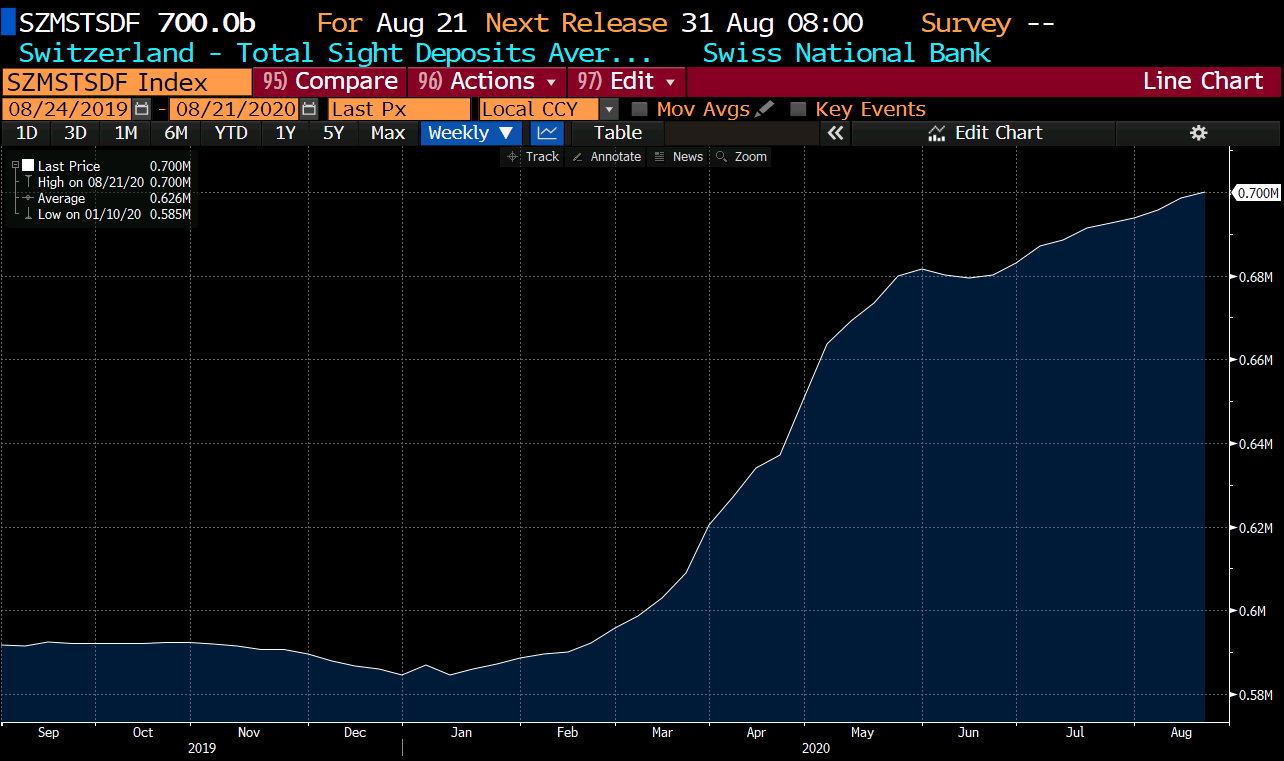A detailed caption for the described image could be:

"This screenshot features a detailed line graph tracking data from September 2019 through to August 2020. The x-axis is labeled with monthly intervals, beginning at September 2019 and progressing through to August 2020. The y-axis scales from 0.58 million to 0.7 million, with incremental markings at 0.58, 0.6, 0.62, 0.64, 0.66, 0.68, and 0.7 million.

At the top of the graph, the label 'SZMSTSDF700B for August 21st' is prominently displayed. The next scheduled release is indicated as "31 August" with the time listed as "8:00 AM." Additional details include a reference to a survey conducted in Switzerland, focusing on "total slight deposits" or possibly "average" deposits, abbreviated as "AVER...".

Further annotations include mentions of the Swiss National Bank, alongside actions like "95 compare," "96 actions," and "97 edit." The type of graph is confirmed as a "line chart.""